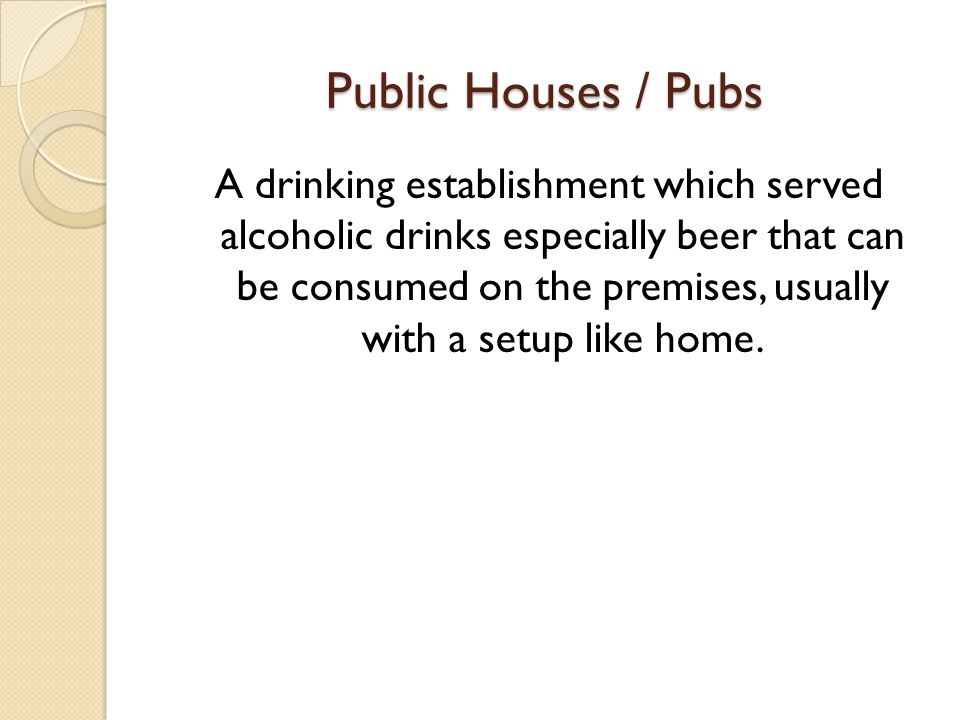The image appears to be a PowerPoint presentation slide with a predominantly white background. On the left side, there's a vertical beige banner adorned with several circles near the top, including one solid beige circle and two circle outlines in white and dark grey beige. The centered heading at the top of the slide reads "Public Houses / Pubs" in a dark brown color. Below this, in black text, is the description "A drinking establishment which served alcoholic drinks, especially beer, that can be consumed on the premises, usually with a setup like Home."